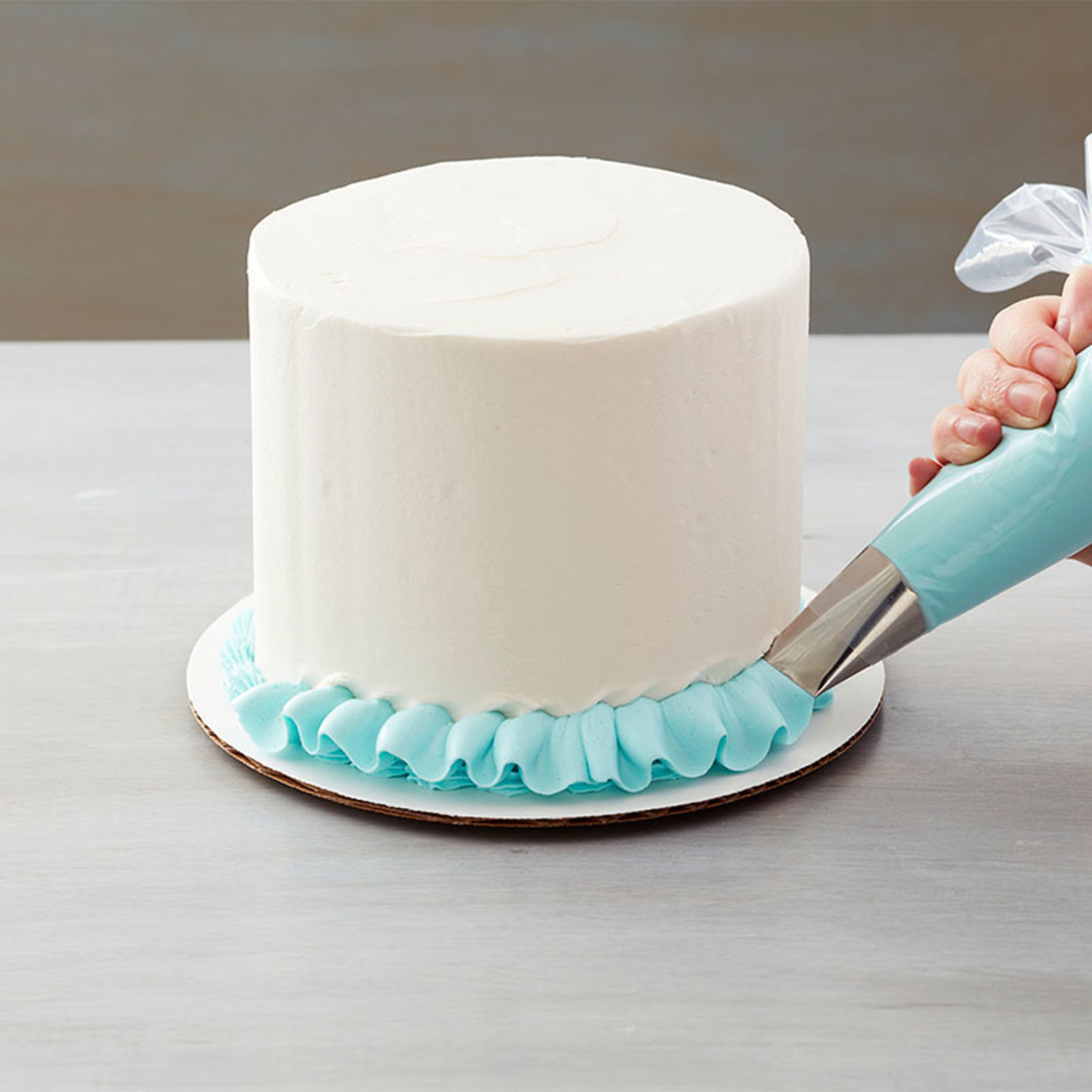The image depicts a white-iced cake resting on a round cardboard base with brown sides, which itself is placed on a gray wooden table. A white hand is seen using a blue piping bag with a silver tip to apply blue frosting in a wavy, ribbon-like pattern around the bottom edge of the cake. The background features a gray wall, and the overall scene suggests that the cake decoration is in progress, with the blue frosting being the only added decoration so far.